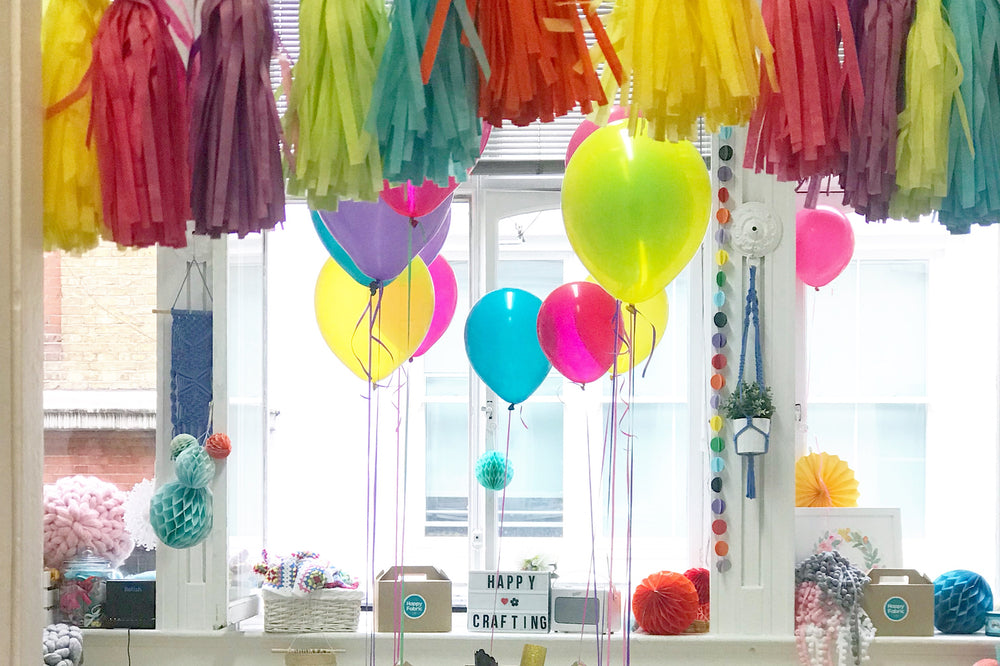The image depicts a bright and colorful room set up for a vibrant crafting celebration, possibly geared towards a birthday party. The elongated horizontal photograph showcases an array of multicolored decorations that immediately catch the eye. Crepe paper streamers in shades of yellow, red, purple, green, dark green, orange, and light blue cascade from the ceiling. Helium-filled balloons, securely tied with strings, float around the room in hues of yellow, pink, blue, green, and purple, adding to the festive atmosphere.

Central to the scene is a table draped in a white tablecloth, prominently displaying a sign that reads "Happy Crafting." The table is adorned with a variety of baskets and containers filled with unknown items likely intended for party activities. Nestled among these are several colorful crepe paper balls and possibly pom-poms, which contribute to the lively setting. On the wall hangs a small succulent plant in a macramé holder, adding a touch of greenery to the space. In the background, a window overlooks a neighboring house, and a door with a large window inset is also visible, contributing to the room's airy ambiance. The combined elements create an inviting and joyful environment perfect for a crafting-themed celebration.